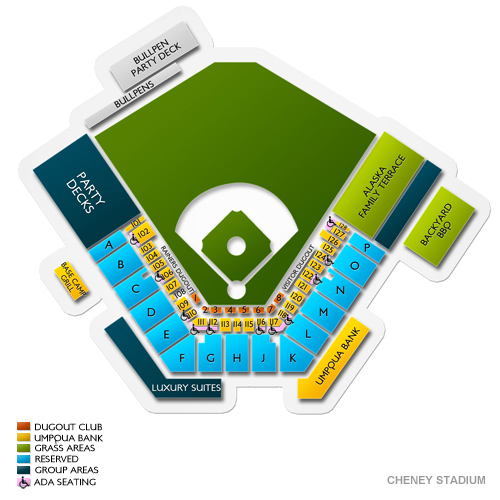Here's a detailed and cleaned-up caption based on the provided information:

---

**Detailed Seating Chart of Cheney Stadium**

This seating chart of Cheney Stadium includes a comprehensive legend and detailed layout. The color-coded legend identifies various seating areas as follows:
- **Dugout Club (Red)**
- **Limb or Umpolia Bank (Yellow)**
- **Grass Area (Green)**
- **Reserved Seating (Blue)**
- **Group Areas (Black)**
- **ADA Seating (Pink with Wheelchair Logo)**

The diagram is structured like a diamond where the top and bottom points are extended to form the green "Grass Area." The infield is depicted in white, with a distinct white circle in the middle representing the pitcher's mound, and another white circle diametrically opposite for the catcher's spot.

Proceeding around the diamond from the upper left corner:
- The **Bullpen** and **Party Deck** are noted first.
- Further along are additional **Bullpens**.
- The **Party Decks** are indicated in dark blue.

The blue "Reserved" section begins with section A and extends downward around the diamond, skirting behind the catcher's position and then back up, ending with the Alaska Family Terrace. A smaller row behind these sections is designated as the **Limb or Umpolia Bank (Yellow)**. 

Beyond this, the **Dugout Club (Red)** occupies its own area. If the diagram is zoomed out, additional features become visible:
- **Base Camp**
- **Grill**
- **Luxury Suites**
- **Backyard Barbecue**

These labels detail the amenities and seating arrangements available at Cheney Stadium, ensuring a clear and informative layout for attendees.